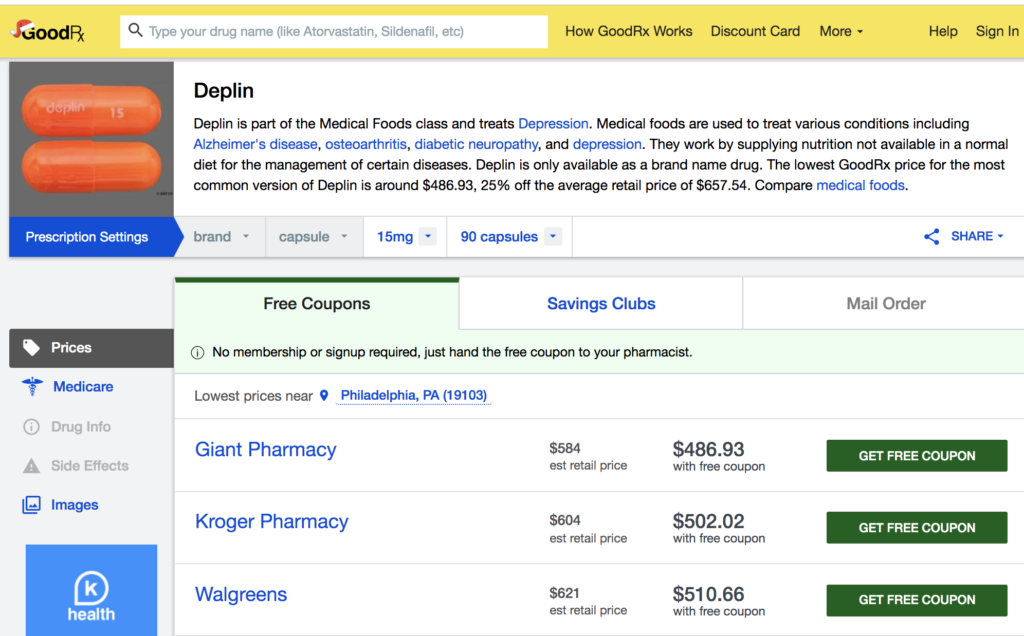The image is a screenshot of the GoodRx website, featuring a prominent yellow bar across the top. On the upper left-hand corner, the GoodRx logo is displayed, with the "G" festively adorned with a Santa hat. Adjacent to the logo is a white text box for users to type in the name of their drug.

Centrally, the navigation menu includes options such as "How GoodRx Works," "Discount Card," "More," "Help," and "Sign In." Below this menu, there is an image on the left side showing two orange pills, accompanied by the label "Deplin" spelled out as "D-E-P-L-I-N." The description clarifies that Deplin is a medical food designed to treat depression.

Directly beneath this section, a blue box titled "Prescription Settings" provides options for the drug. It displays selections for "Brand," "Capsule," with "15 milligrams" and "90 capsules" chosen via drop-down menus.

To the right of this section, a link symbol followed by the word "Share" is present. Below, three tabs are visible: "Free Coupons" (which is highlighted), "Savings Clubs," and "Mail Order." Under "Free Coupons," it mentions, "No membership or sign-up required, just hand the coupon to your pharmacist." The lowest prices are specified for location "Philadelphia, Pennsylvania, 19103," and the three chosen pharmacies are Giant Pharmacy, Kroger Pharmacy, and Walgreens.

Beneath the image of the orange pills on the left, another menu bar includes options like "Prices," "Medicare," "Drug Info," "Side Effects," and "Images." At the very bottom, a blue box features a "K" inside a raindrop-like shape, accompanied by the word "Health."